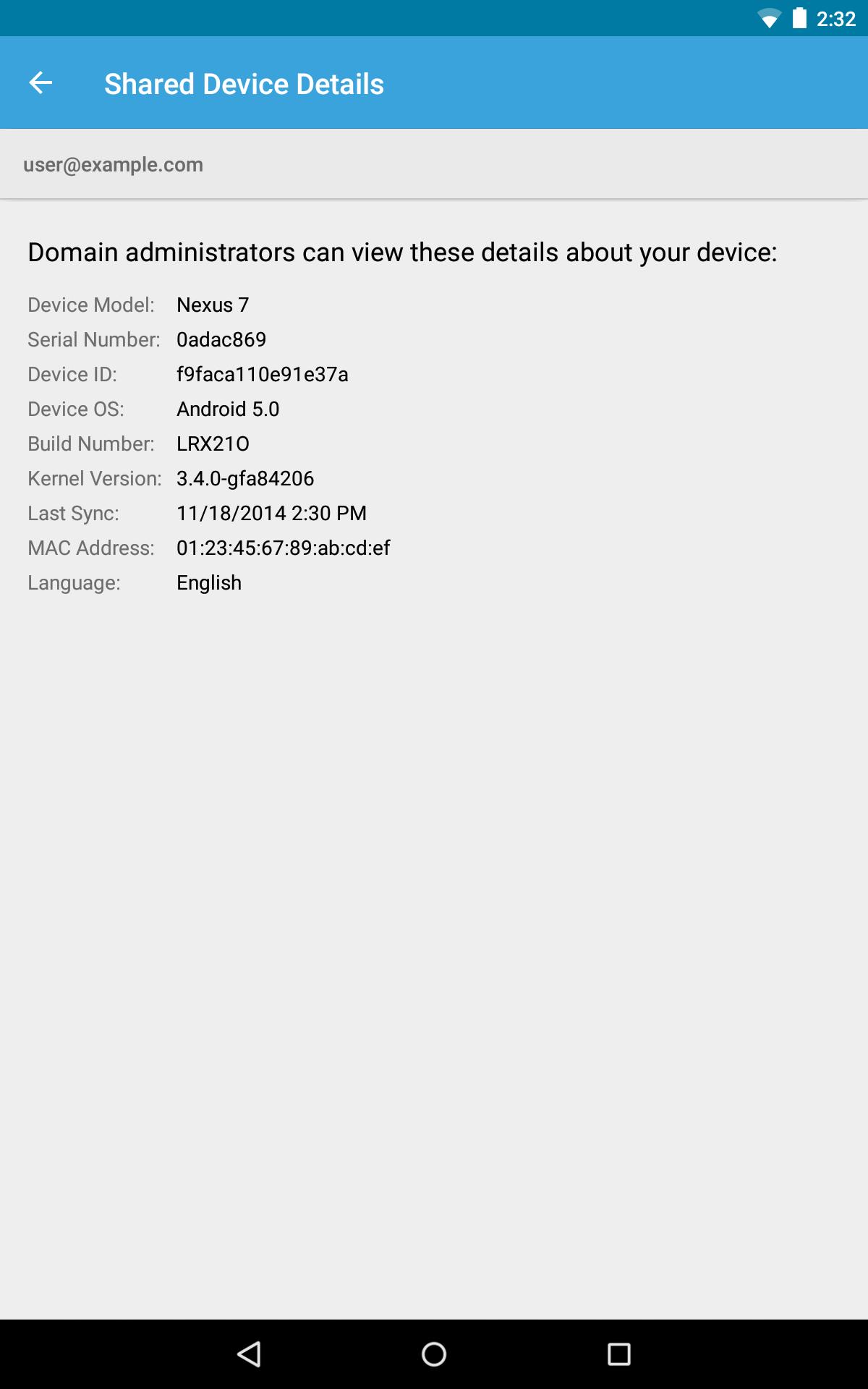Here is a detailed caption for the image:

---

This image displays detailed information about a shared device, specifically a Nexus 7 tablet. The device is registered under the user email "user@example.com." Domain administrators have the capability to view the following details:

- **Device Model:** Nexus 7
- **Serial Number:** 0ADAC869
- **Device ID:** F9FACALL0E91E37A
- **Operating System:** Android 5
- **Build Number:** LRX210
- **Kernel Version:** 3.40 GFA84206
- **Last Synced:** November 18, 2014, at 2:30 PM
- **MAC Address:** 0123456789ABCDEF
- **Language Settings:** English

At the bottom of the screen, a black strip displays additional controls for the phone or tablet.